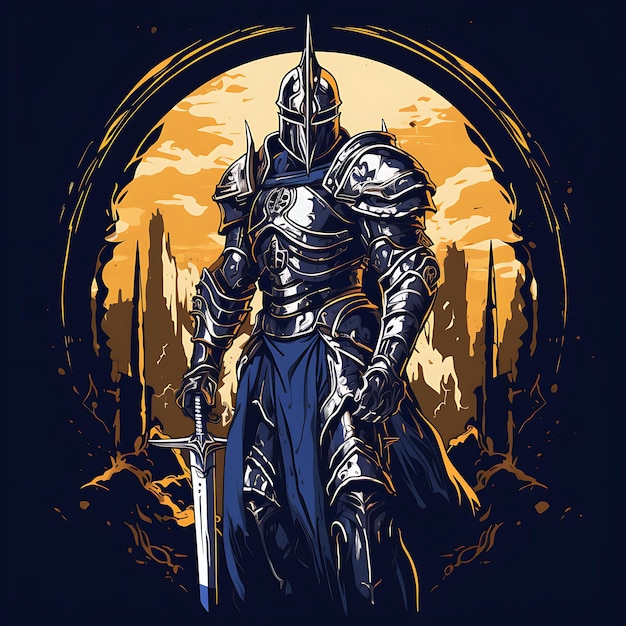The image is a detailed digital illustration of a knight, rendered in a comic style. The knight, clad in reflective silver armor accented with blue cloth, stands heroically in a centralized position against a dramatic mountainous backdrop formed by a circular frame, reminiscent of a cave entrance. His face is obscured by a large, pointed helmet featuring small rectangular slits for eyes and a prominent metal blade running down its length. He holds a sword in his right hand, the blade of which is directed downward. The background reveals a desolate, fantasy landscape with a sky that transitions from orange to yellow hues, suggesting a setting sun. Decorative accents, including pointy elements and circles, embellish his armor, contributing to his imposing and possibly villainous stature. The overall aesthetic and graphical details suggest that this image could be from a video game.